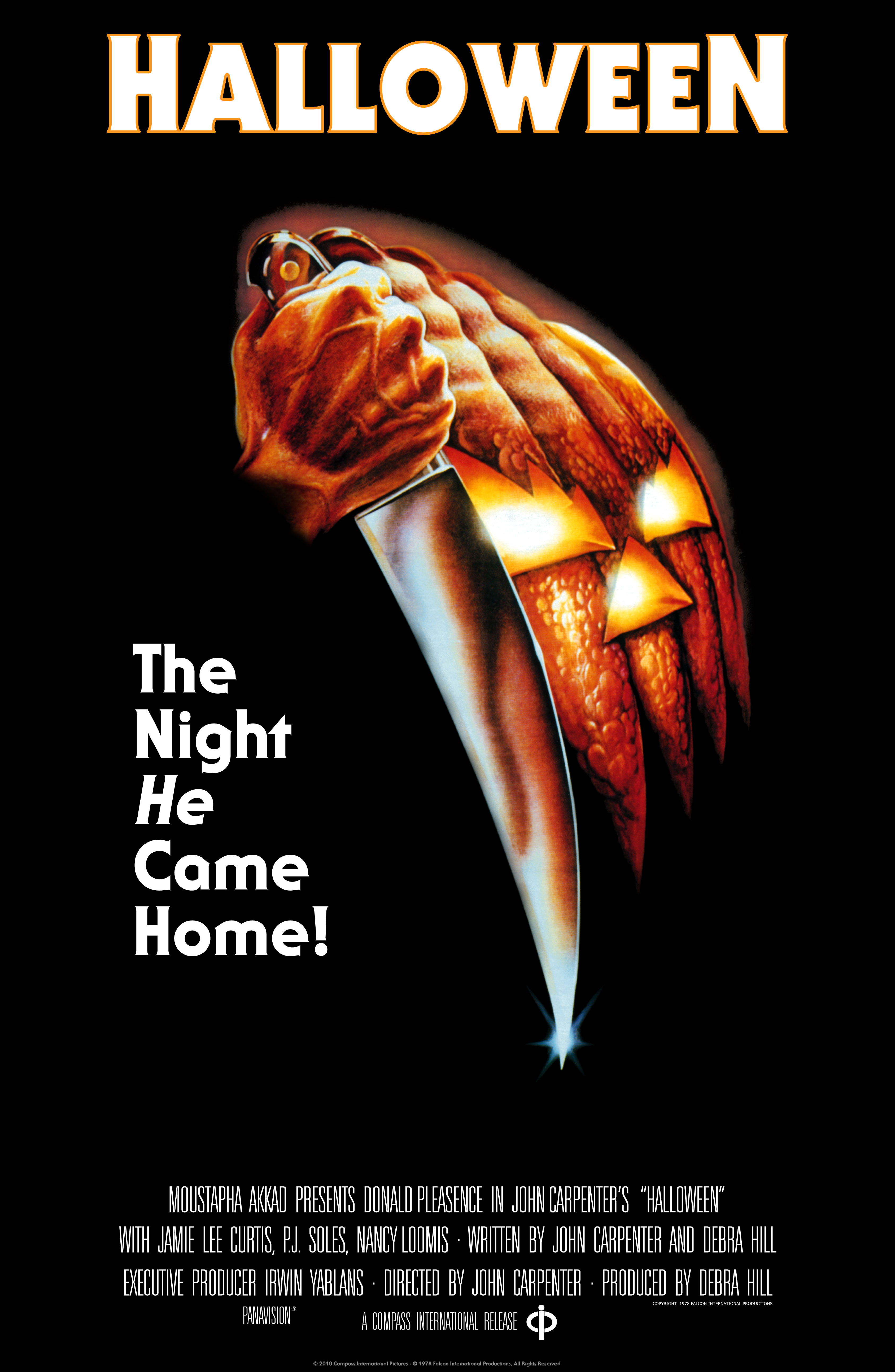This is a classic movie poster for John Carpenter's iconic horror film, "Halloween," featuring a deep, black background. Dominating the top of the poster is the movie title, "Halloween," rendered in bold, white letters. Below the title, a menacing illustration emerges: a hand, seemingly carved from a pumpkin with veined, orange knuckles resembling claws, tightly grasps a long, curved, silver knife. The knife's metallic blade catches the light, sparkling at its sharp tip. This hand appears to be part of a jack-o'-lantern face, which looms ominously behind it. The face is carved into an orange pumpkin, complete with triangular eyes and nose, glowing with a yellowish hue as if illuminated by an internal flame. Beside this eerie image, the phrase "The night he came home" appears in white letters on the left side. The bottom of the poster features additional text, listing the names of the cast and crew involved in the making of the film, all set against the black background.